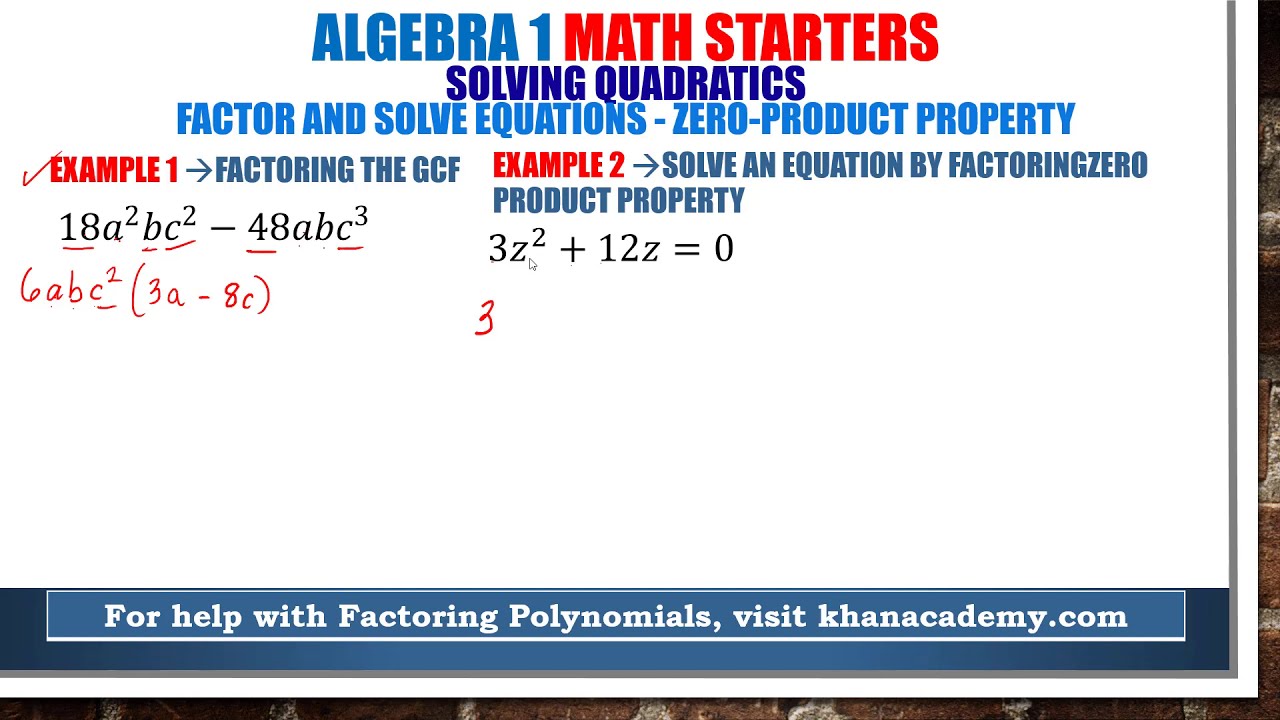The image is a screenshot likely from an educational resource, such as Khan Academy, designed to help with Algebra 1 math problems. The white background features various text elements in different shades of blue and red. At the top, "Algebra 1" is written in blue, followed by "Math Starters" in red. Beneath that, "Solving Quadratics" appears in darker blue, under which "Factor and Solve Equations - Zero Product Property" is displayed in lighter blue. The image includes mathematical examples: the first example is labeled "Factoring the GCF" with a corresponding equation, and the second example is "Solve the Equation by Factoring - Zero Product Property" with another equation. At the bottom, there is a blue banner with white text that reads, "For help with factoring polynomials, visit khanacademy.com." The overall style resembles an instructional ad or educational aid commonly used for learning algebra concepts.